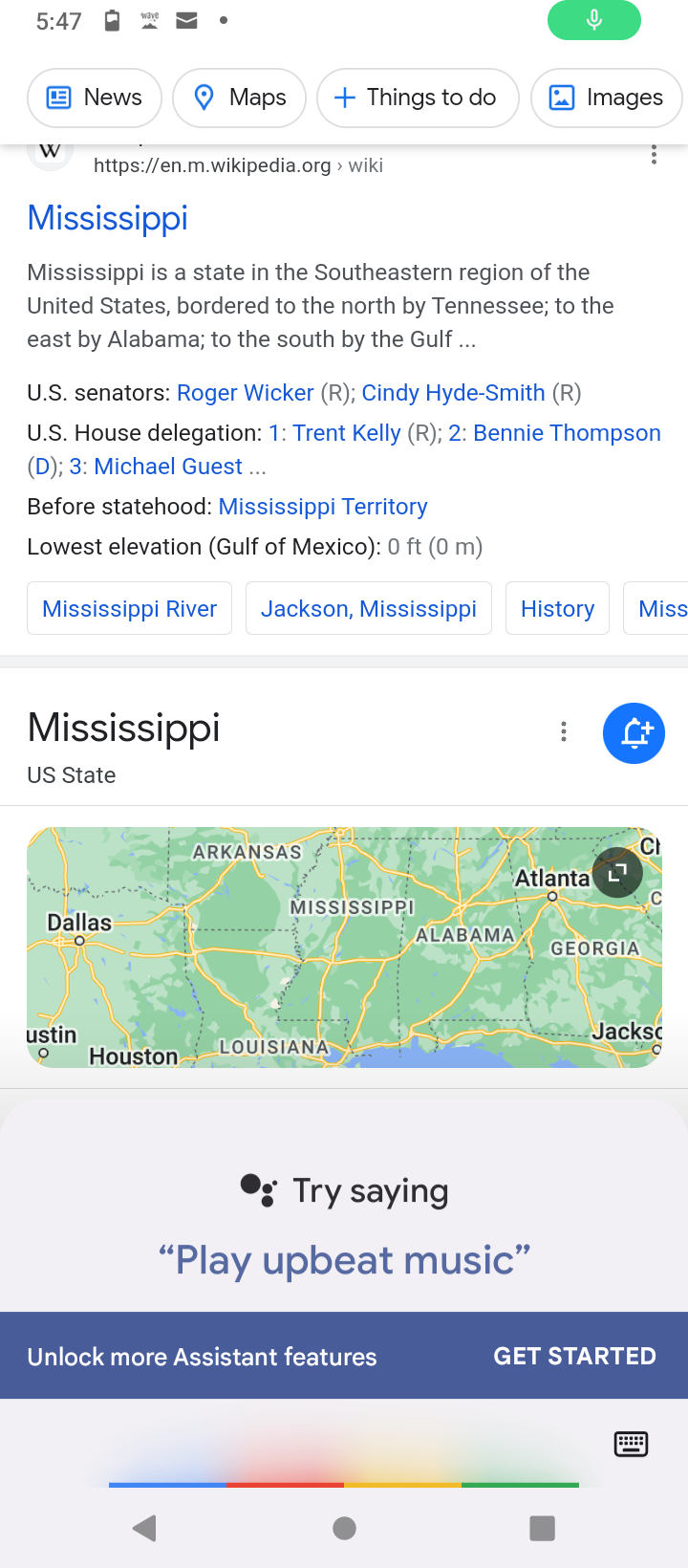The image is a detailed screenshot of a smartphone, captured in portrait mode. It appears to depict results from a search for "Mississippi" on Google Chrome, showcasing the Wikipedia page for Mississippi at the top. The upper left corner of the screen shows the time as 5:47 and indicates the phone is about half charged. Various icons are visible, including a battery icon, a WAVE icon, and an envelope. To the right, a microphone icon is displayed within a green oval circle. Below, navigation options like "news," "maps," "things to do," and "images" are visible.

The main content shows detailed information about Mississippi, including its statehood, geography, and location in the southeastern United States, bordered by states like Tennessee and Alabama. A colorful map is featured beneath this text, rendered in varying shades of green to possibly indicate elevation, and displaying major cities such as Jacksonville, Atlanta, Houston, Austin, and Dallas—although these cities are not within Mississippi.

Below the map, there's an ad banner with the message "try saying play upbeat music" and instructions to "unlock more assistant features" by clicking "get started," highlighted by a colorful line running across the bottom with segments in blue, red, yellow, and green.